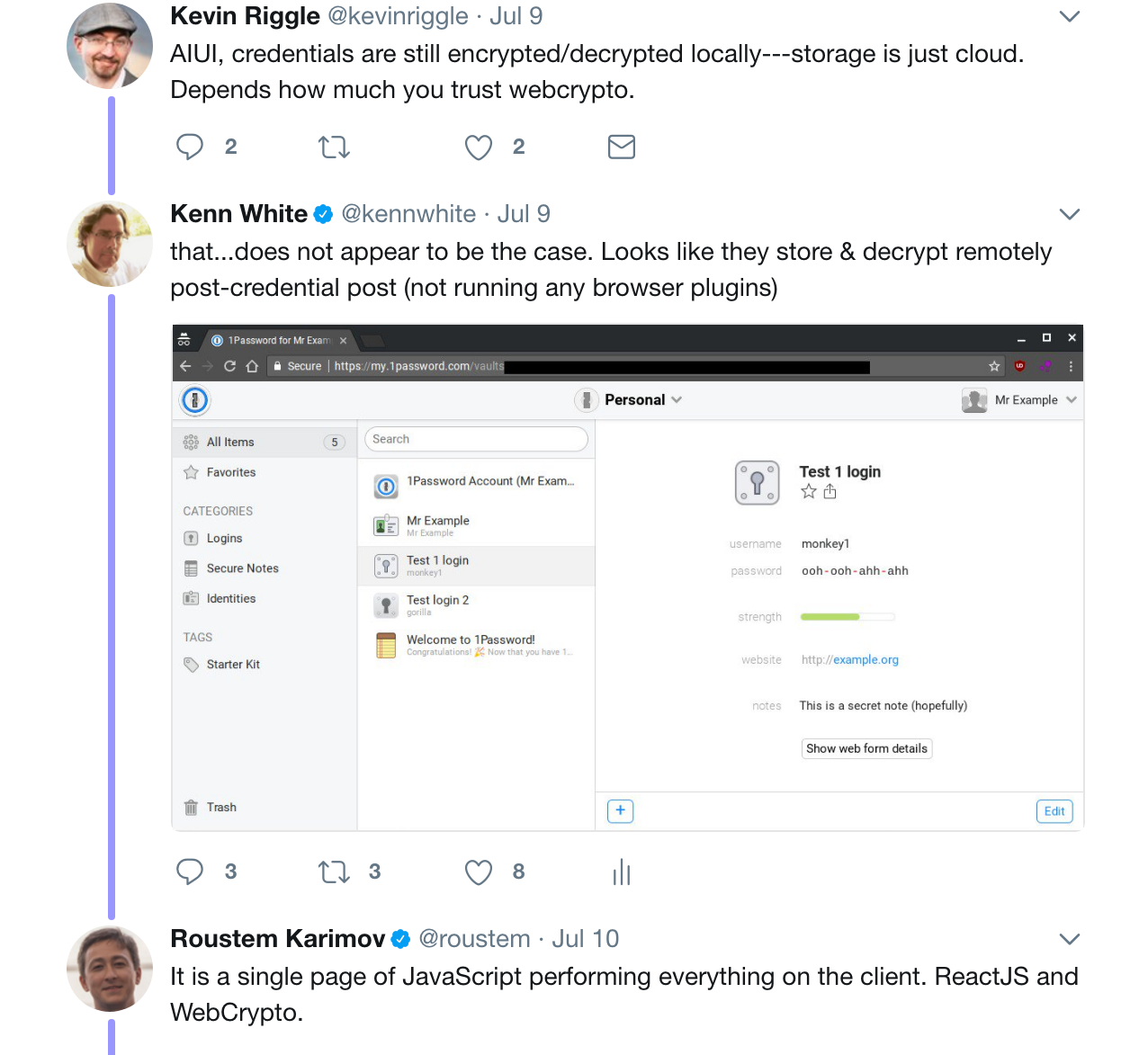This image depicts a lively conversation on social media, centered around the technical details of how a website manages login information. The vertical orientation of the image suggests it could be a screenshot taken either from a computer or a mobile device. The background is stark white, highlighting the string of posts and replies.

In the top-left corner, there is a circular profile picture of a man. He bears a driver's cap and glasses, along with a goatee. This is Kevin Riggle, whose handle is @KevinRiggle. On July 9, Kevin posted, "AI UI credentials are still encrypted, decrypted locally. Storage is just cloud. Depends how much you trust web crypto."

Right beneath Kevin's post, another user, Ken White (with the handle @KenWhite), responded also on July 9. Ken's reply includes a skeptical comment: "... does not appear to be the case. Looks like they store and decrypt remotely post-credential post (not running any browser plug-ins)." Accompanying Ken's post is a screenshot of a web browser, presumably serving as evidence to support his claim.

The conversation continues with Rustam Karabov (@Rustam), who posted on July 10: "It is a single page of JavaScript performing everything on the client, React.js and web crypto." 

This dialogue captures the nuances of a technical debate over the methods employed by a particular website in handling login credentials, with participants scrutinizing the security and implementation details using industry-specific jargon.